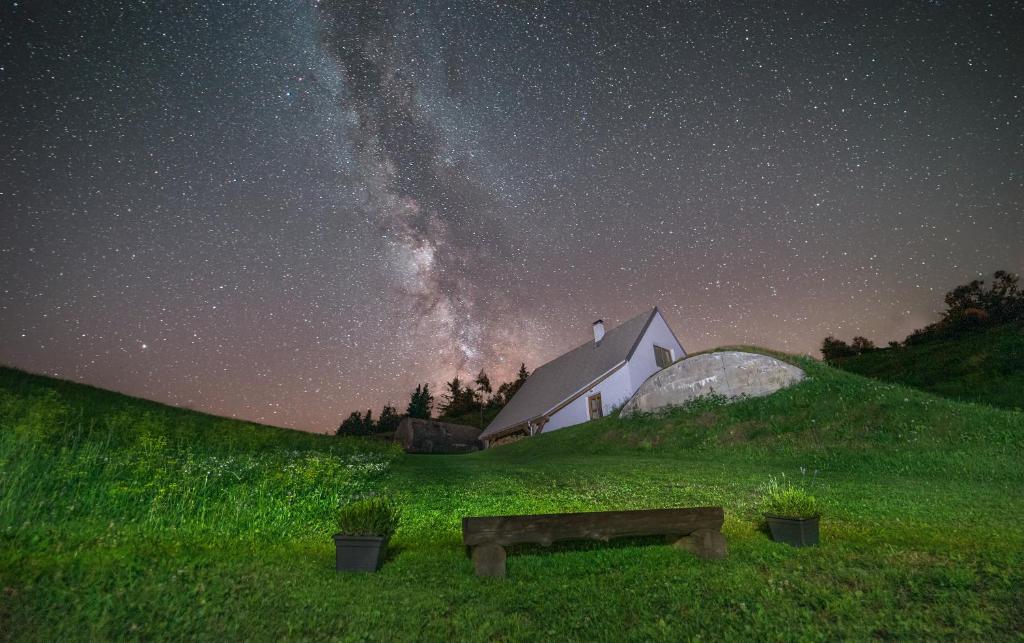The image captures a breathtaking nighttime scene where the vast, starlit sky dominates the upper two-thirds of the photograph. Highlighted by the brilliance of the Milky Way and hints of the Northern Lights, the night sky gradually transitions from deep black at the top to a warm orangish hue near the horizon, reflecting the final moments of a sunset. Below this celestial display, a white A-frame house with a gray roof sits atop a gently rolling hill, accompanied by a few trees on either side. The house features a small chimney, and the area around it includes smoke suggesting a recent event. In the foreground, vibrant green grass spreads out, interrupted by a wooden bench with half-log design, flanked by two black plant holders containing small plants. On the right side, a low stone wall adds an element of rustic charm to the scene. The photograph combines both the natural beauty of the night sky with a serene, homely atmosphere, capturing the tranquil transition from day to night.